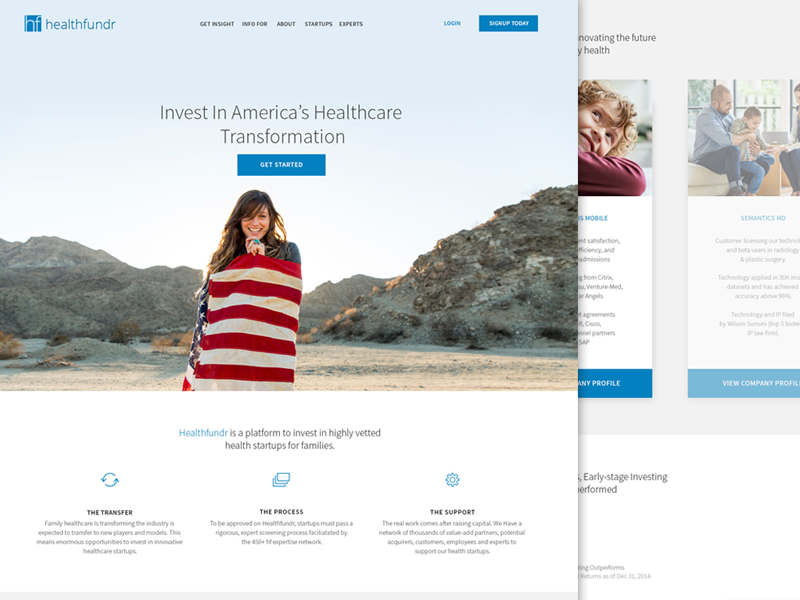The image captures the homepage of the Health Funder website. Prominently displayed in the upper left corner is the "HF" logo, with "Health Funder" spelled out beside it. The background of the webpage features a striking visual of a desert-like mountainous area with brown dirt or sand. In the center of this background, a woman stands wrapped in an American flag. Above her, the text reads, "Invest in America's healthcare transformation," accompanied by a "Get Started" button.

In the upper center portion of the page, navigation options include tabs labeled "Get Insight," "Info," "Startups," and "Expert." The upper right corner features "Login" and "Sign Up Today" buttons, facilitating user access.

The bottom half of the image transitions to a white background where it states, "Health Funder is a platform to invest in highly vetted health startups for families." Below this explanatory text, there are three sections: 
1. "The Transfer" - offering relevant information.
2. "The Process" - outlining procedural details.
3. "The Support" - containing a paragraph of supportive text.

This detailed composition effectively communicates the mission and offerings of the Health Funder platform.